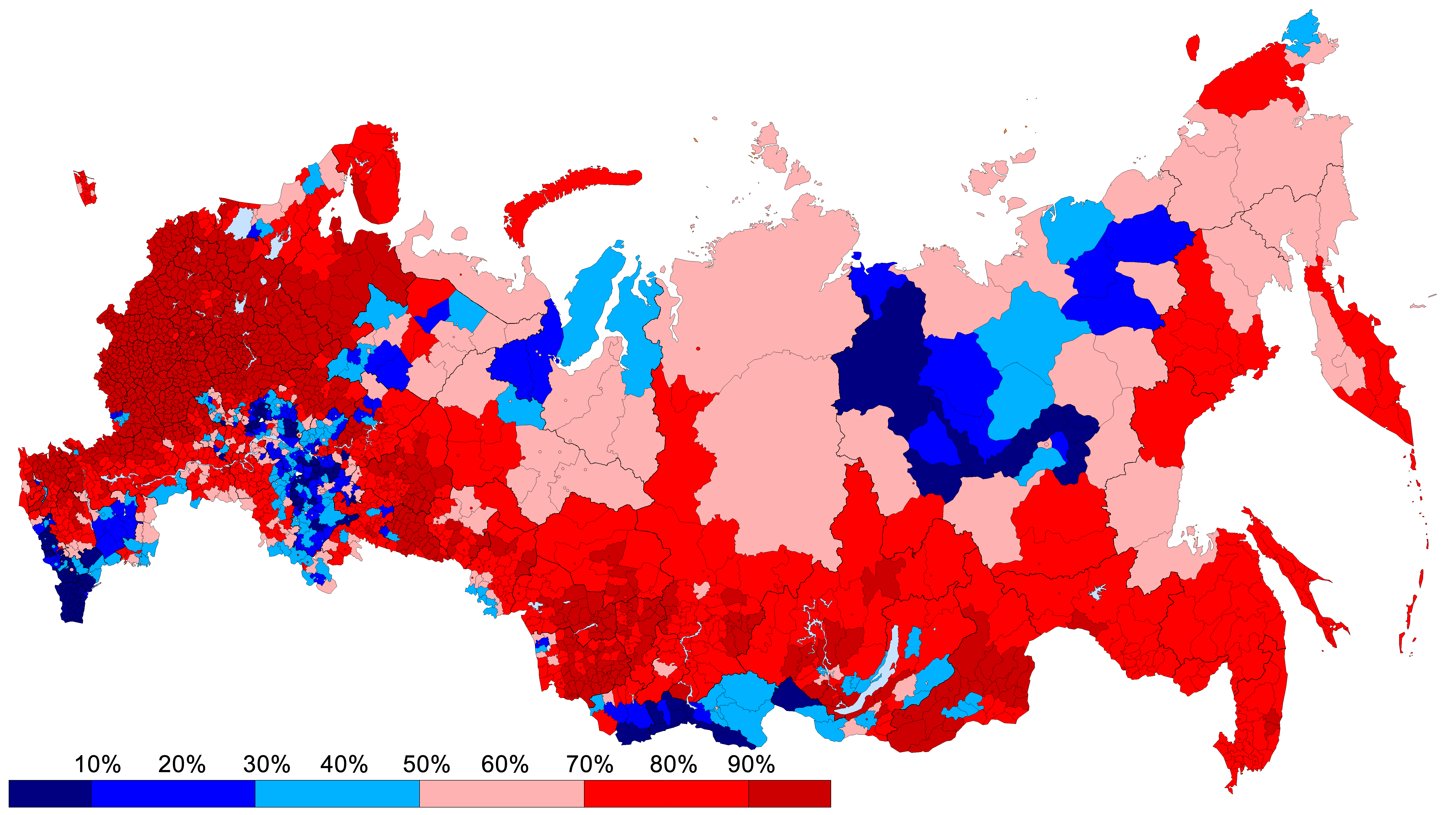This detailed photograph depicts a country divided into numerous small regions, each distinctly color-coded according to a gradient legend displayed at the bottom. The legend ranges from deep blue (almost black) indicating 0%, to dark red representing 100%. The entire country is a mosaic of these colors, with each county or political subdivision illustrated in varying hues. These areas vary significantly in size; some regions are large while others are relatively small.

The geographic shape of the country bears a resemblance to a running dog, sprinting from right to left. Central regions predominantly feature a pinkish hue, indicating a 60% value of the measured parameter. On the leftmost edge, areas are marked by dark red, signifying they fall within the 90% to 100% range of the specified measurement.

Additionally, at the bottom of the map, there are regions marked in deep red, highlighting 100% measurements. Despite this, the map exhibits an overall balanced mix of blues, reds, and pinks, creating a visually diverse and detailed representation of the data being illustrated. The exact geographical identity remains unclear, though it distinctly differs from Europe and bears some resemblance to Russia.